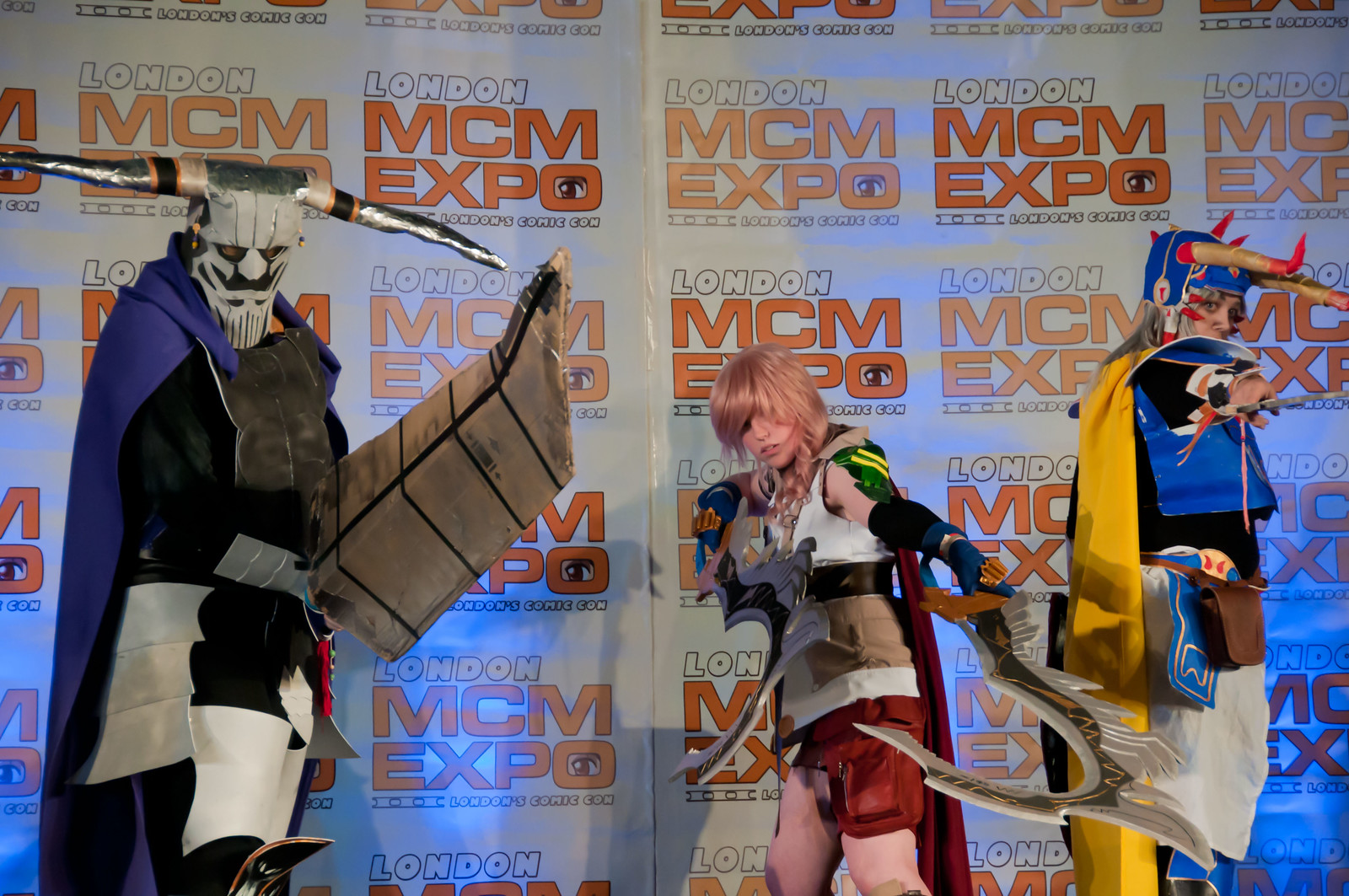This vibrant photograph captures a trio of cosplayers at the London MCM Expo, an event akin to Comic-Con, as evidenced by the repeating "London MCM Expo" posters in the backdrop. On the left stands a figure in an elaborate costume: a white mask adorned with silver horns and a purple hooded cape over a predominantly black outfit, complete with a wing and possibly a large sword or shield. The central character is a girl with striking blonde hair, dressed in black gloves, a sleeveless belted shirt, and vivid red shorts. She wields two long, hook-like weapons and strikes a dynamic fighting pose. Completing the ensemble on the right, a gentleman sports a distinctive blue horned helmet with brown horns, a yellow cape, a blue vest, and white pants. This detailed tableau brings to life the creativity and spirit of the cosplay community at the expo.